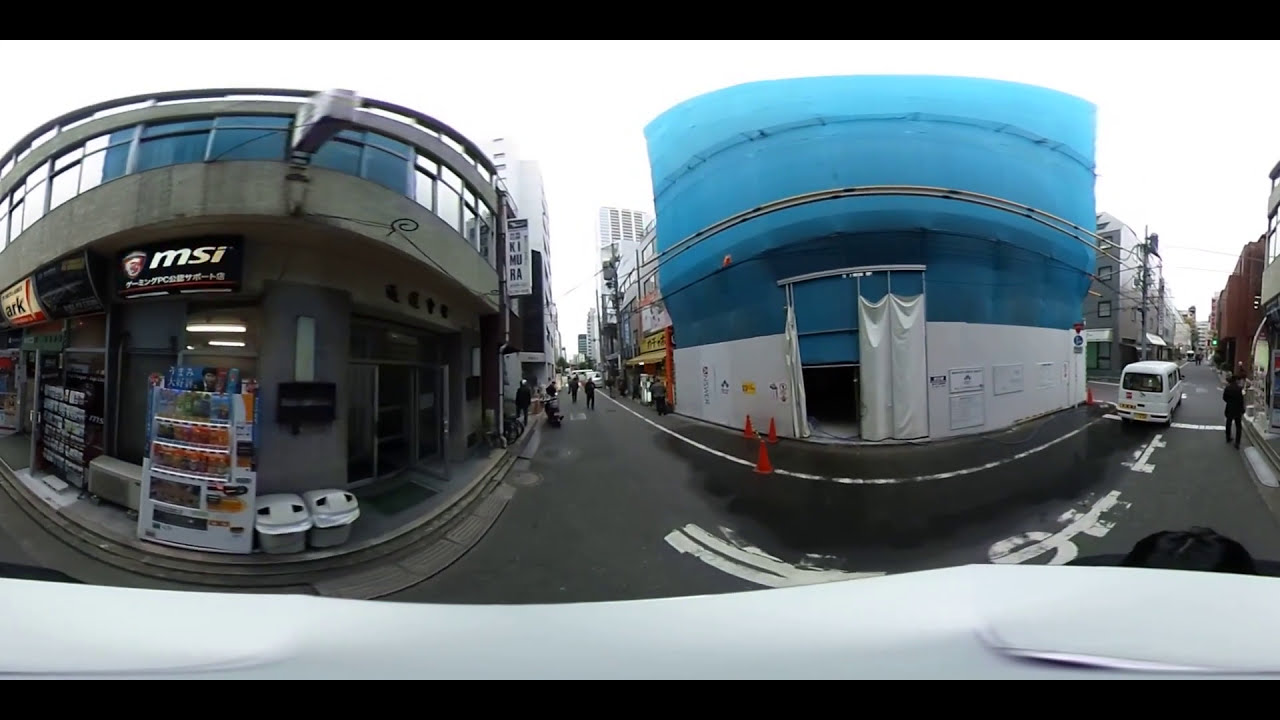This is a panoramic cityscape image with a distinct swirling and looping effect, capturing a bustling urban street. The composition is centered around two main structures: a building with a blue roof and an open garage on the right, and a cluster of small, connected stores on the left, resembling hole-in-the-wall shops. The scene is set on a narrow street, flanked by these buildings. 

Towards the right, a white van or car is seen driving away, with cones marking an entrance to a building. In the middle of the image, a few tiny figures walk away from the camera, dressed predominantly in black. Notably, there's a shop sign featuring "MSI" and a stand displaying bottles, sodas, and various goods for sale, enhancing the lively atmosphere of the scene.

The sky is bright and white, casting a day-lit ambience over the area. Power lines on poles dot the street, which showcases elements suggestive of a foreign country, possibly Asian, as indicated by the letters on the storefronts. There's also a hanging curtain or blanket in front of a garage door on the right side. The lower half of the image slightly resembles the hood of a white car, adding to the city's busy, layered vibe.